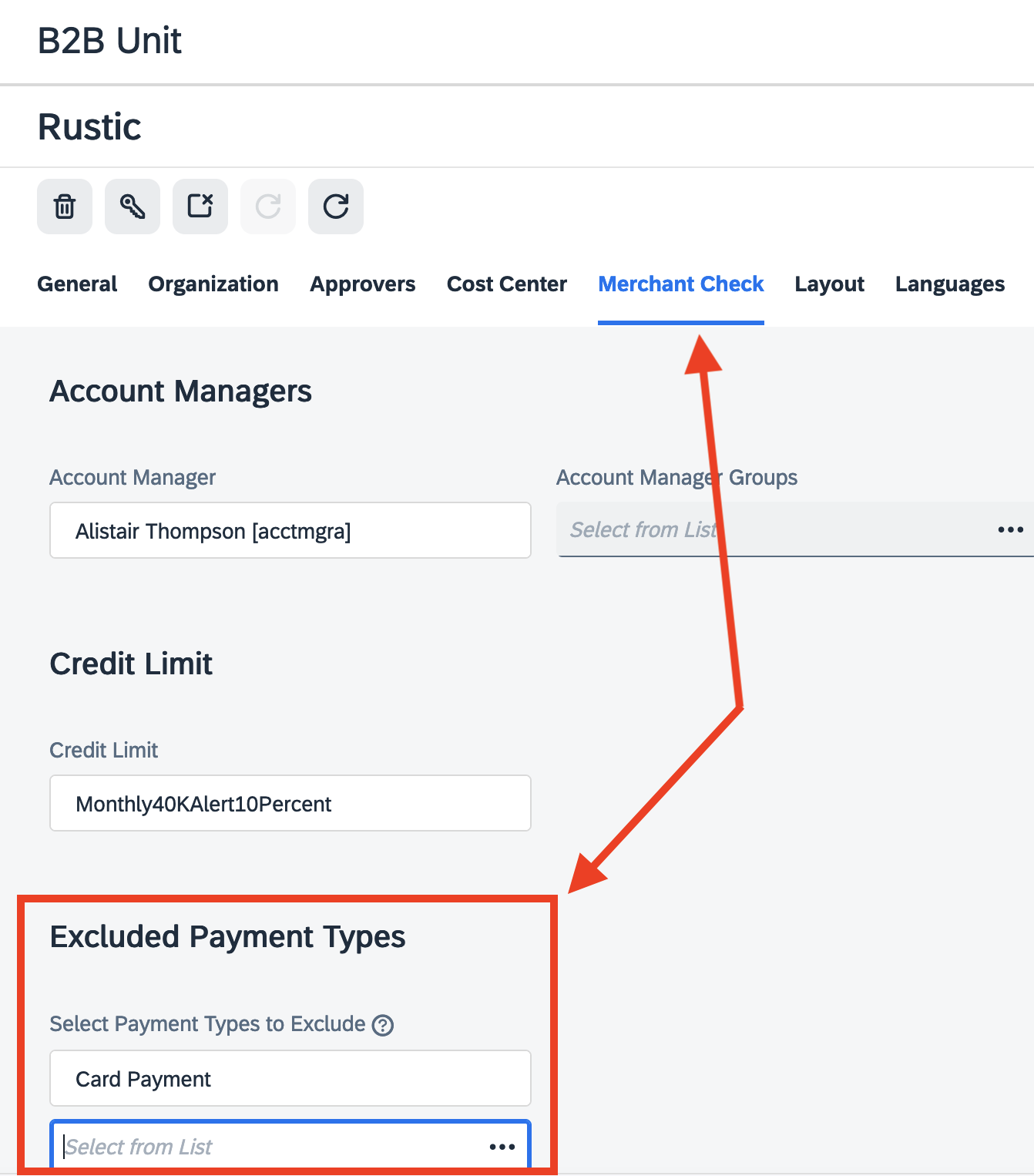**Screenshot Description:**

This screenshot captures a detailed configuration page within a financial or management software platform, identified at the top as "B2B unit" under the subsection "Rustic".

**Visual Elements:**

- **Top Section:**
  - On the upper left, the "B2B unit" and "Rustic" labels are prominently displayed.
  - A series of icons includes:
    - A trash can icon
    - A key icon
    - A square icon with an 'X' in the upper right-hand corner
    - A grayed-out icon resembling a circular arrow
    - A similar circular arrow icon that is fully colored and clickable.

- **Navigation Menu:**
  - Below, a list of categories is present, such as "General", "Organization", "Approvers", "Cost Center", "Merchant Check", "Layout", and "Languages".
  - The "Merchant Check" category is highlighted in blue, indicating it is currently selected; others remain in black.

- **Main Configuration Area:**
  - **Top Section Details:**
    - Text in this area includes "Account Managers" in a primary font with "account manager" repeated below in gray.
    - The name "Alastair Thompson" is listed as an account manager (abbreviated as "ACT, ACCT, MGRA" in parentheses).
  - **To the Right:**
    - "Account Manager Groups" fill a section with a "Select from List" field nearby, accompanied by three dots, but it is currently unfilled.
  - **Lower Section Details:**
    - "Credit Limit" is highlighted twice, once in a prominent font and again in a smaller gray font.
    - The associated search box includes terms: "Monthly 40K Alert 10%".
  - **Highlighted Red Box:**
    - Located at the bottom left, outlined in red, labeled "Excluded Payment Types".
    - Instructions "Select payment types to exclude" are displayed with a question mark icon for help.
    - The search box within is populated with "Card payment".
  
- **Additional Interface Elements:**
  - Another input field below the red box; labeled "Select from list", outlined in blue.
  - Two arrows present:
    - One pointing downwards towards the blue-bordered box
    - Another pointing straight up towards the "Merchant Check" blue-highlighted category.

This extensive layout addresses account management, payment exclusions, and various financial configurations, featuring dynamic elements like search boxes, selection lists, and actionable icons for user interaction.